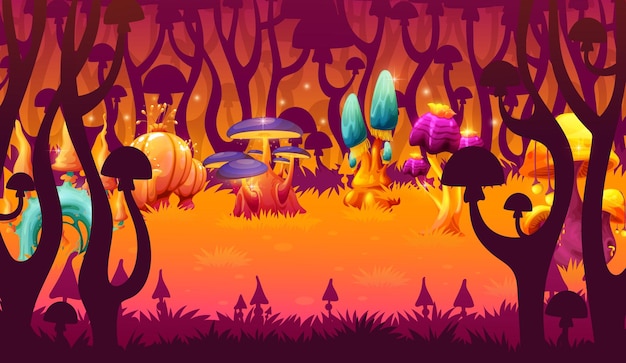The illustration is a magical and vibrant mushroom kingdom depicted in a cartoonish, animated style. At the center, there's an open meadow, or glade, illuminated in bright and vivid hues like blues, purples, teals, pinks, and golds. The meadow is populated by an array of stylized mushrooms with colors spanning from purple to aqua, dark purple, orange, and yellow. Some have blue tops, while others display a variety of shapes, including oval and umbrella-like forms. These mushrooms, growing from what resemble thicker stalks or mounds, dominate the foreground.

Surrounding this central meadow, the scene transitions into a forest where the vegetation continues the mushroom motif. The trees, both in the foreground and distant background, are dark silhouettes crowned with mushroom-like shapes, suggesting an enchanted woodland. The grassy terrain varies in color from golden and pinkish hues to orangish shades, enhancing the otherworldly ambiance.

The background gradient features a mix of pink, orange, and yellow, shifting to darker shades towards the foreground, adding depth to the digital artwork. Tiny mushrooms dot the landscape, contributing to the lively, magical atmosphere. Overall, the illustration exudes a playful and bright surrealism, creating a visually captivating scene.